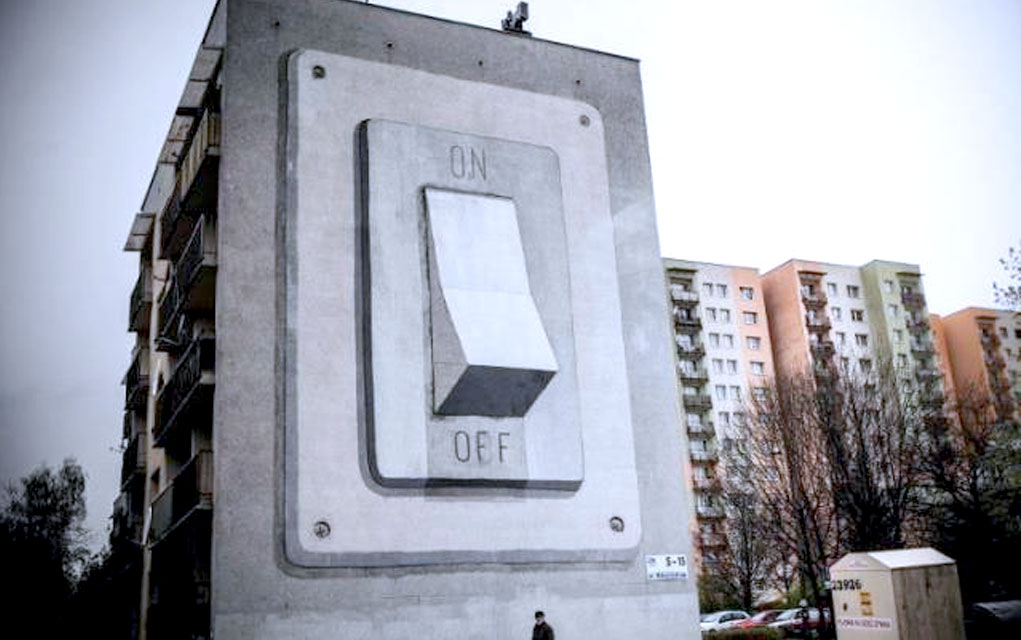The image depicts a close-up, multi-story gray building, approximately 4-5 floors high, with a detailed 3D-like 2D painting of an on-off switch on its side. The painted switch has "ON" at the top and "OFF" at the bottom, and the artwork's realistic coloring and shading create an illusion of depth making the switch appear almost tangible. The painted switch covers about three floors of the building. In the background, there are additional buildings, likely apartment complexes or hotels, standing around 15-16 stories tall, with a light orange tint. The scene includes wintery leafless trees, cars, and what appears to be a small shed in the lower right. At the base of the main building, a real person stands, barely visible, adding scale to the overall mural. The main colors in the image are shades of white and gray, enhancing the striking contrast of the painted switch.